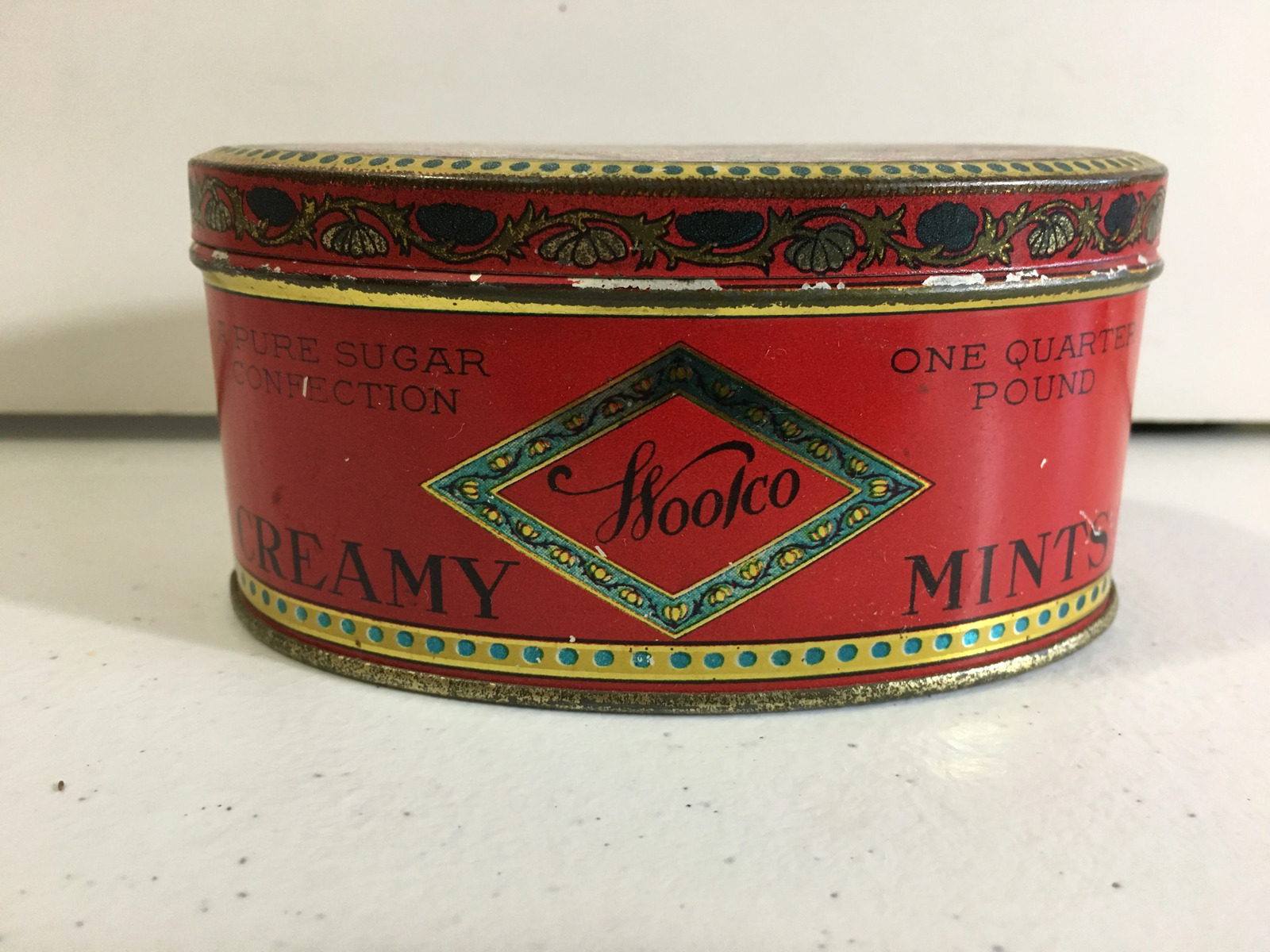An antique tin container of creamy mints is depicted in this photograph. The tin, predominantly red with gold and green highlights and intricate floral designs, features a meticulously detailed central diamond-shaped logo. The logo, which appears to read "WUKU," is surrounded by a border resembling flowers and vines, consistent with the decorative motif along the top of the container. The tin bears the inscription "creamy mints" in bold black lettering on the lower left and right sections, with "pure sugar confection" on the left and "one quarter pound" on the right. Gold trim with evenly spaced blue circles adorns the bottom edge of the container. It sits on a marbled surface with a white wall as the backdrop, further emphasizing its classic, nostalgic appeal.